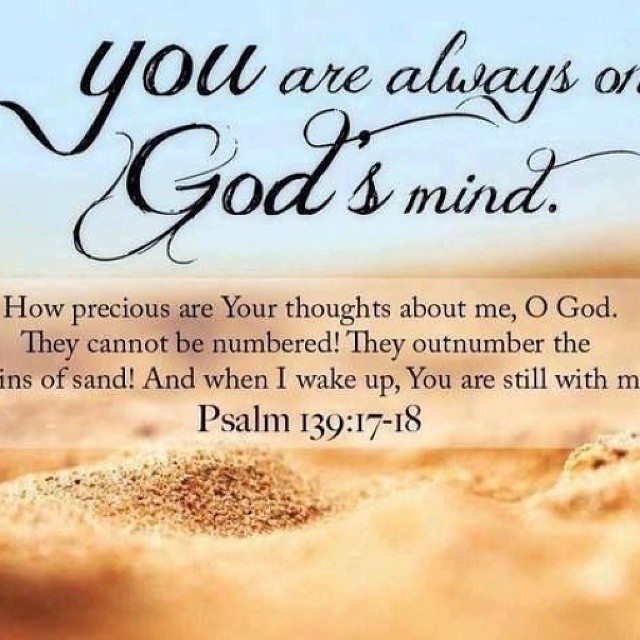This square, color photograph merges photographic representationalism with graphic design. The upper half showcases a pale blue sky, and the lower portion displays a sandy surface, resembling a serene beach scene. At the top, in elegant black cursive, it reads, “You are always on God's mind,” though some letters are cut off at the edges. Below this, in a horizontal rectangular section with black typewritten font against the sand, the text states: “How precious are your thoughts about me, Oh God. They cannot be numbered! They outnumber the grains of sand! And when I wake up, you are still with me.” Below this inspirational message, the scripture is cited as “Psalm 139:17-18,” emphasizing the spiritual nature. The overall composition suggests tranquility and divine reflection, though the full verse and some script details are partially cut off.